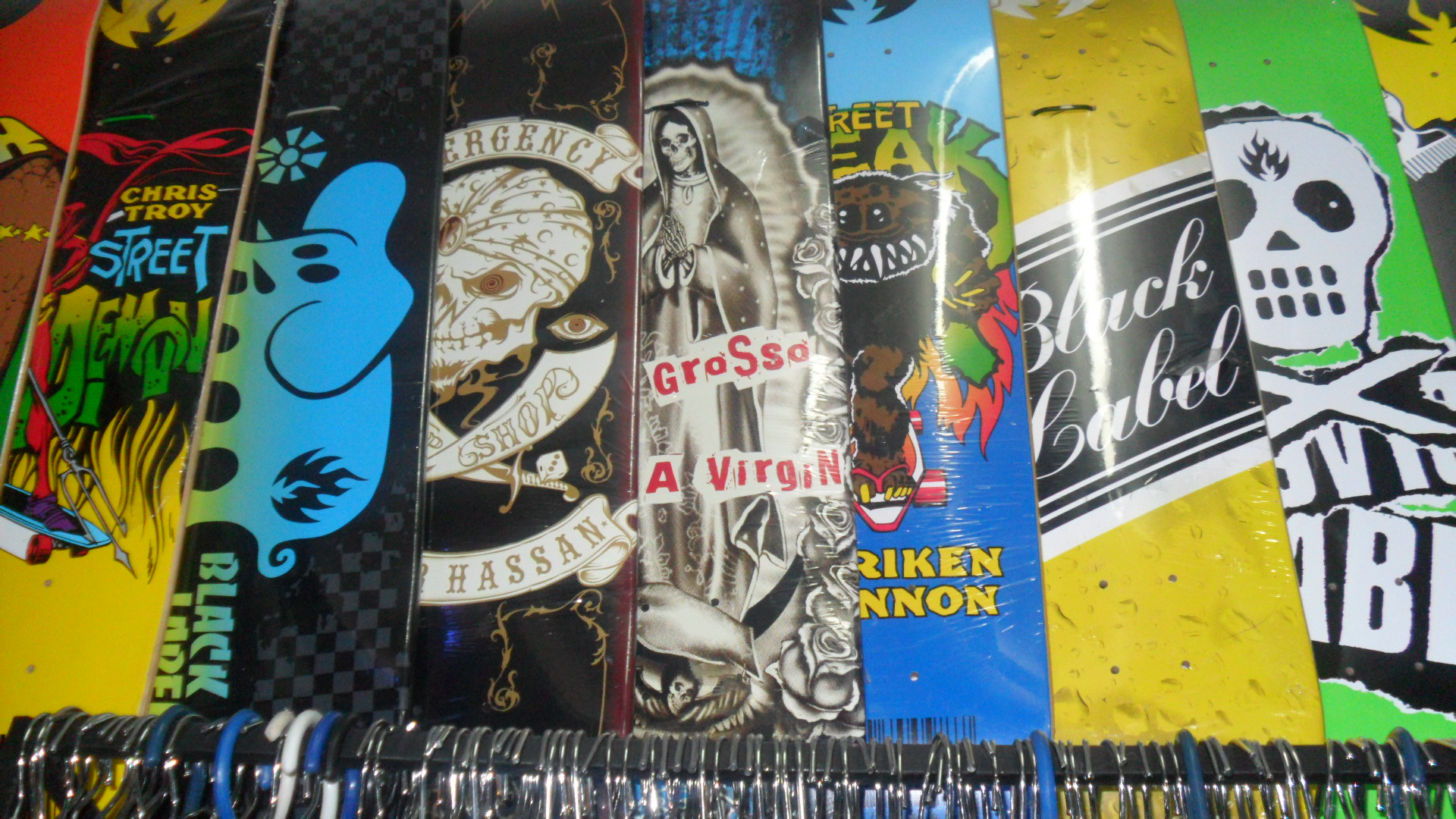The image showcases a close-up view inside a clothing store, where attention is drawn to a row of garment hangers on a black bar at the bottom of the frame. The hangers are predominantly silver-toned with a few plastic ones interspersed, but the clothing items themselves are obscured. In the background, a series of vibrant, overlapping plastic skateboards or banners is visible. They feature diverse and colorful designs, creating a rich tapestry of artwork. Some of the notable elements include:

1. **Chris Troy Street Poster**: A black skateboard with deep green and red lettering.
2. **Black Label Banner**: Characterized by a yellow and black color scheme with white lettering and black stripes.
3. **Grasa A Virgin Poster**: Featuring a hooded skeleton in a grayish robe, encircled by a light blue gradient with red text.
4. **Skull with Headband and Jewel**: A black background with white inscription "Emergency" and accompanied by a sword and an eyeball graphic.
5. **Blue Elephant Design**: Presented against checkered gray and black, the elephant gazes at a blue flower with black flames in the background.
6. **Monster with Long Fangs**: Displaying a red background with yellow and black details and the partially legible inscription "reet, eek."
7. **Hockey Mask Graphic**: Shown with a green background and black eyes, featuring a central flame and white Xs.

The intricate and animated backdrop, suggesting a fusion of both skateboarding and clothing culture, adds a dynamic and eclectic atmosphere to the store.